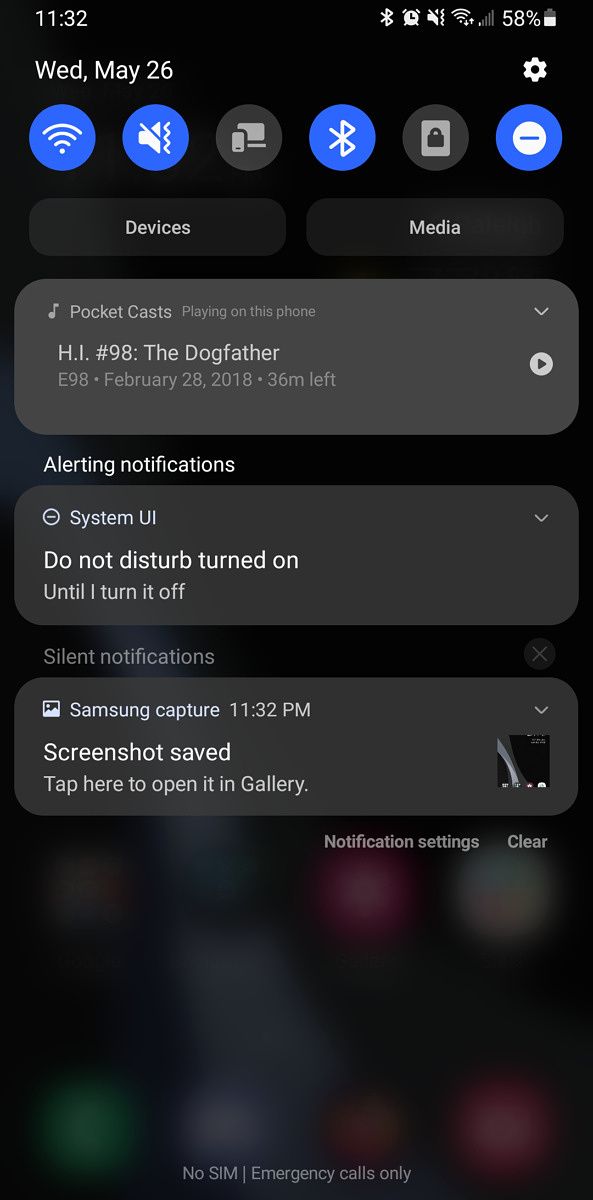### Notification Screen on a Smartphone

**Screenshot Timestamp:** 11:32 PM (Top-left corner)
- **Icons (Top-right corner):** 
  - Bluetooth icon
  - Alarm clock icon
  - Sound turned off icon
  - Strong Wi-Fi signal (one bar)
  - Regular signal (one bar)
  - Battery life (58%)

**Icons Repeated:**
- In circles at the top of the notification screen, including a lock icon and a circle with a bar inside it.

**Buttons:**
- **Devices**
- **Media**

**Notification Panels:** 
- **Alerting Notifications:**
  - _"Plucky Cast Playing on This Phone"_
    - H1 Number 98: The Dog Father Episode 98
    - Date: February 20th, 2018
    - Time Left: 36 minutes
  - _System UI: Do Not Disturb On_
    - Subtext: "Until I turn it off"
  
- **Silent Notifications:**
  - _Samsung Capture at 11:32 PM_
    - Subtext: "Screenshot saved. Tap here to open the gallery."

Behind these notifications, there is a blurred home screen with various icons. 
The notifications are displayed on lighter gray panels with rounded corners.

**Visual Elements:**
- The blurred home screen and the round icon design create a modern and clean look on the notification screen.